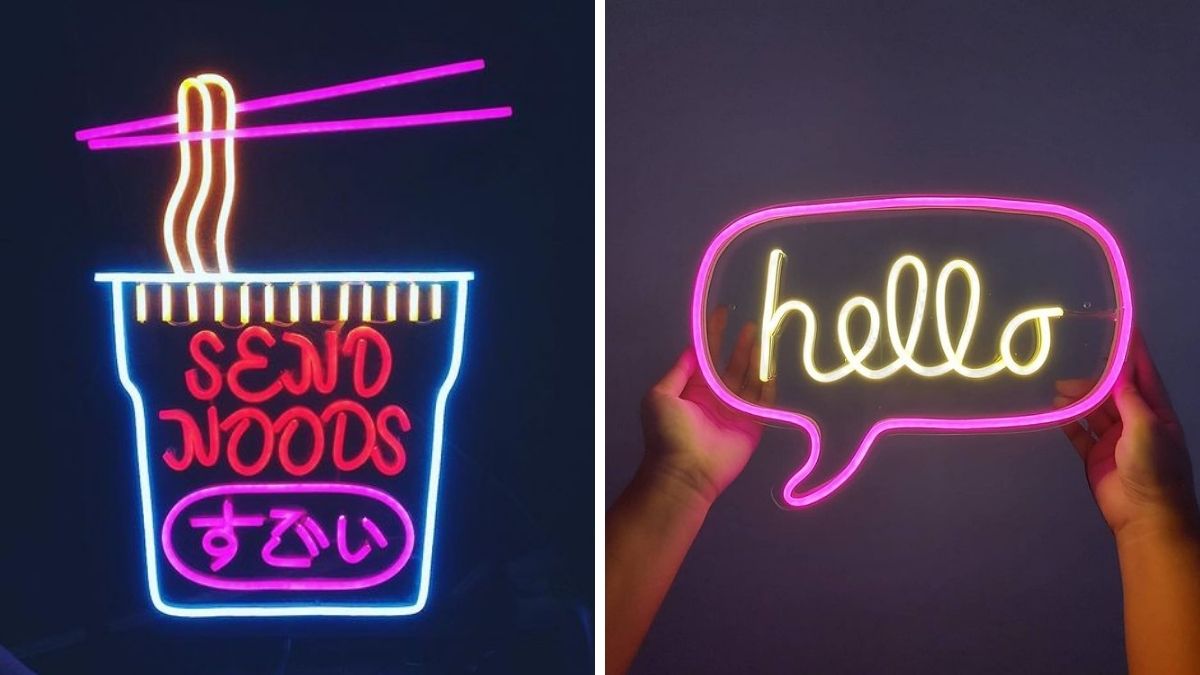The photograph features two vibrant neon signs set against contrasting backgrounds. On the left, a dark blue backdrop highlights a playful neon advertisement depicting a cup of noodle soup. Purple chopsticks lift a cascade of long noodles from the cup, which is adorned with the phrase "Send Noods" in striking red neon and accompanied by Asian characters in matching purple. On the right, against a dark gray background, two white neon hands hold a bright pink neon speech bubble, resembling a comic strip quotation bubble. Inside the bubble, the word "hello" is elegantly written in cursive yellow neon, creating a warm and inviting glow.